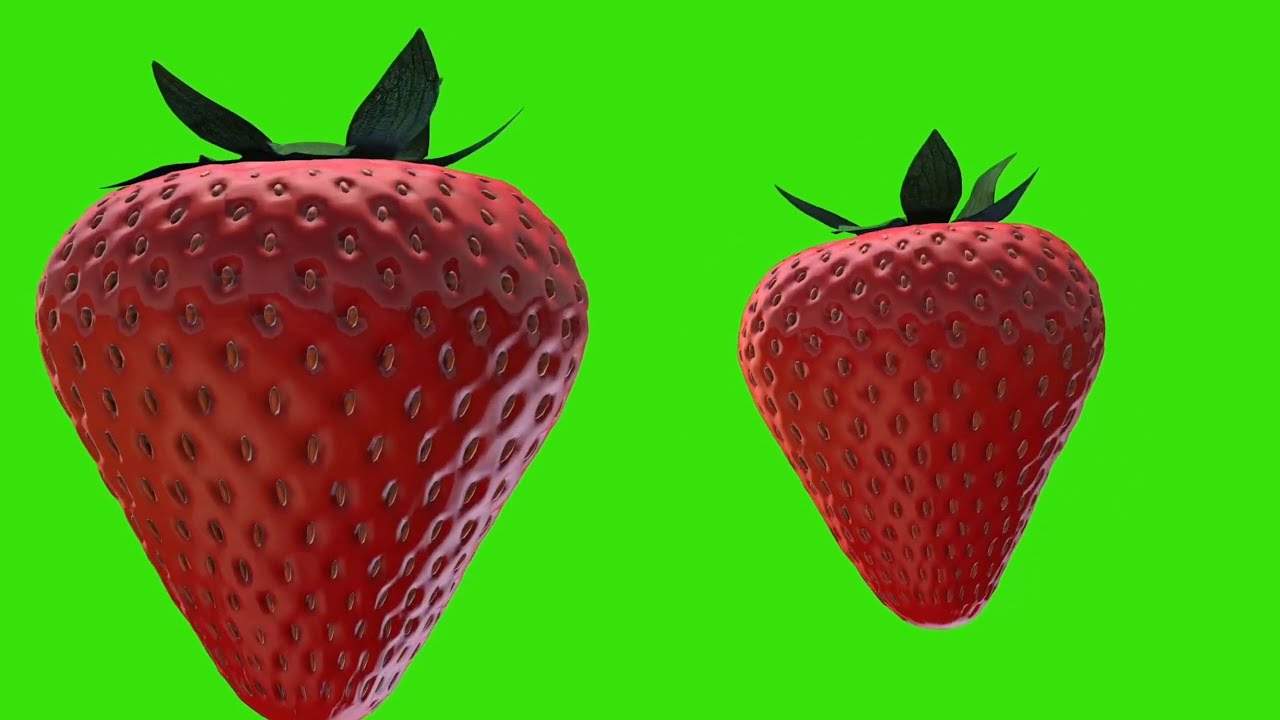The image depicts a simplistic, digital render of two strawberries set against a neon green background, reminiscent of a chroma key screen. The larger strawberry is positioned on the left, slightly cut off at the bottom, and the smaller one is on the right. Both strawberries exhibit a matte yet subtly glowy finish, transitioning from deep red to a lighter red towards the top, creating a sensation as if they've been dipped in water. Detailed with numerous seeds and green leafy stems, the lighting on the left strawberry comes from the top and right, whereas the lighting on the smaller right strawberry is primarily from the top. The background is uniformly lime green, giving a minimalist and vibrant contrast to the red strawberries.